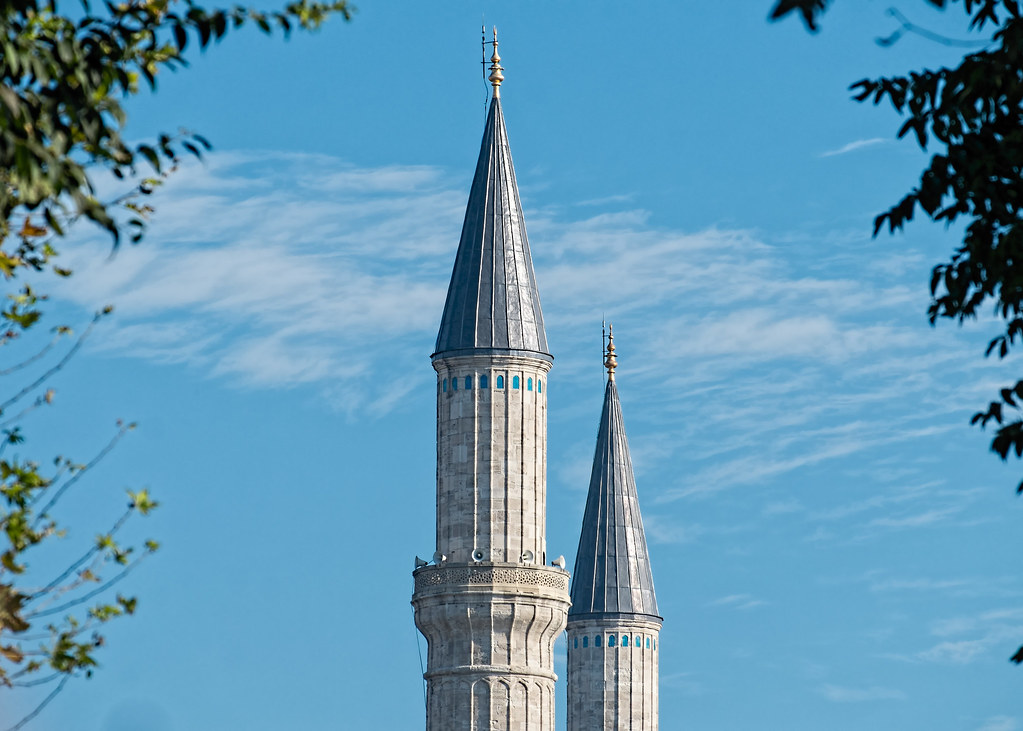The image is a detailed color photograph showcasing the tops of two castle-like spires. The spires, constructed from light gray stone that shows signs of weathering, have windows just below where they transition into cone-shaped, shiny gray tops. The conical sections are adorned with small, brassy embellishments. Vibrant blue windows are situated at the very peak of the stonework, just before the cones begin. The spires are set against a backdrop of a very blue sky with some clouds, flanked by the green crowns of nearby trees.